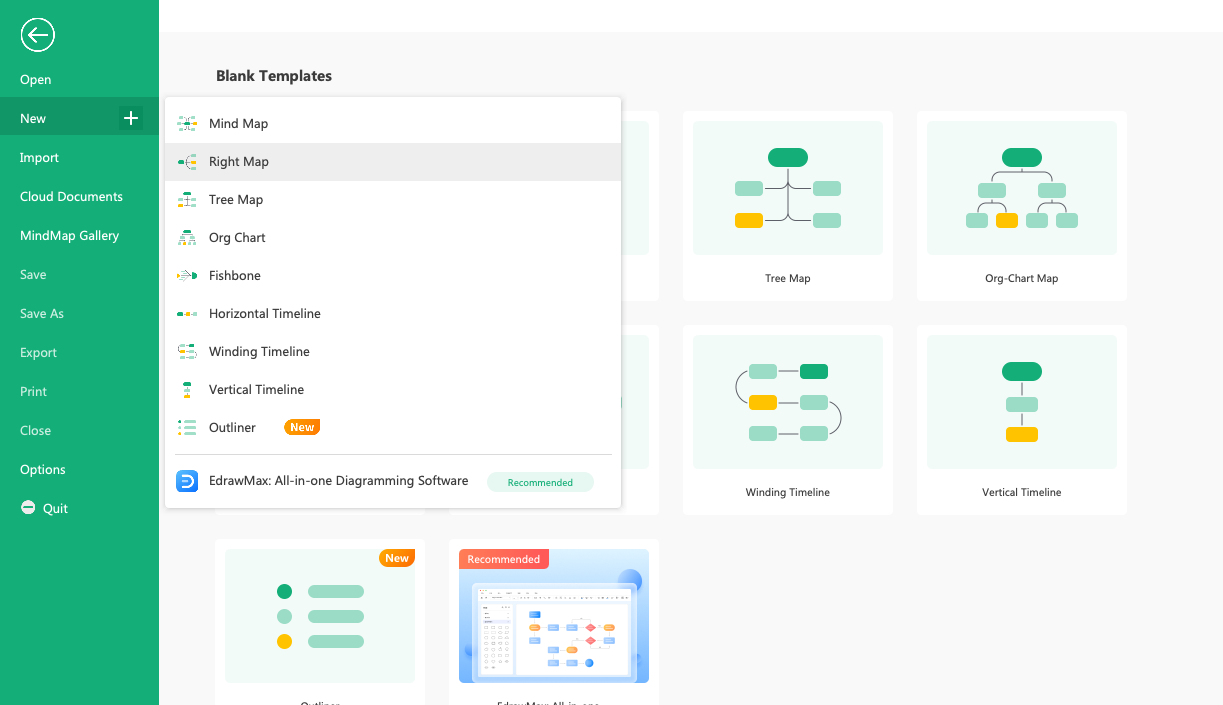The image showcases an application's interface consisting of two primary sections. 

### Left Panel:
- **Background Color**: Green and white, interspersed with blue, red, and orange elements.
- **Iconography & Text**:
    - A circle with an arrow labeled "Open". 
    - A highlighted "New" option with a plus sign.
    - Additional options include "Import", "Cloud Documents", and "Mind Map Gallery".
    - Functional commands such as "Save", "Save As", "Export", "Print", "Close", and "Options".
    - A circle with a bar labeled "Quit".

### Right Panel:
- **Background Color**: Predominantly white.
- **Text**:
    - A header titled "Blank Templates".
    - Lists various template options such as "Mind Map", "Right Map", "Tree Map", "Org Chart", "Fishbone", "Horizontal Timeline", "Winding Timeline", "Vertical Timeline", and "Outliner" (highlighted with the word "New" in orange).
- **Image Preview**:
    - At the bottom, there is a square, blue-framed section titled "Recommended".
    - It displays various chart outlines in green, light green, and orange.

### Additional Details:
- On the right-most side of the image, there are visual depictions of template options like "Tree Map", "Org Chart Map", "Winding Timeline", and "Vertical Timeline", providing a more illustrative view of each category.

This detailed layout gives a comprehensive overview of the application’s user interface, highlighting both navigation options and template previews.